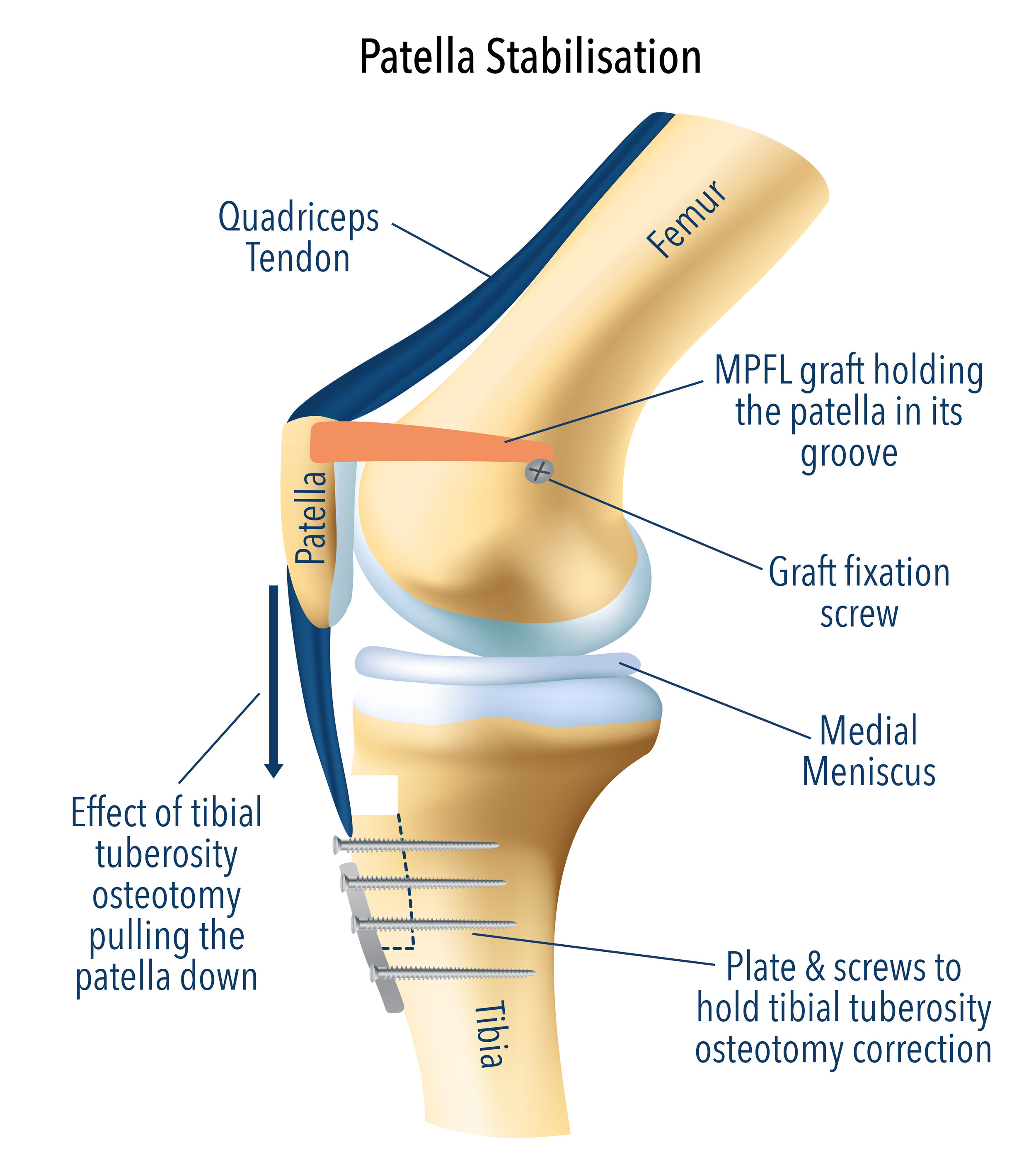This detailed colored illustration depicts a labeled diagram of the skeleton bones and joints of the knee, focusing on patella stabilization. Prominently, the femur (the upper leg bone), the patella (the kneecap), and the tibia (the lower leg bone) are illustrated and clearly labeled. The image outlines the quadriceps tendon located above the femur, indicating its positioning and relationship to the other knee structures.

Significant attention is given to the tibial tuberosity osteotomy, highlighting the procedure’s effect of pulling the patella downwards. Essential elements of this surgical intervention are detailed, including the plates and screws used to secure the tibia post-osteotomy correction. The medial meniscus, situated between the femur and tibia, is also labeled, outlining its critical placement within the knee joint.

Furthermore, the MPFL (Medial Patellofemoral Ligament) graft is shown holding the patella in its groove, as well as the graft fixation screw, emphasizing their roles in the stabilization process. This image serves as an educational resource, suitable for a medical textbook, providing an in-depth look at the anatomical structures and surgical components involved in knee stabilization and potential replacements.